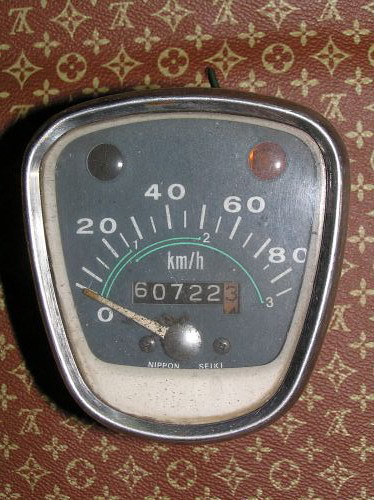This color photograph features a close-up view of a small, antique analog speedometer, likely extracted from a vintage car. The speedometer takes on a distinctive shield-like shape, being slightly wider at the top than at the bottom. It is set within an elegant frame of what appears to be either vinyl or leather, characterized by a medium to light brown hue. Encircling the speedometer are intricate gold motifs, including repeating patterns of four-pointed stars and clovers, which add a refined touch to the overall aesthetic.

The face of the speedometer is a muted gray color, prominently displaying the numbers 20, 40, 60, and 80 around its perimeter. The gauge needle rests at zero, positioned on the far left. At the center of the dial, the odometer registers a mileage of 60,722, further hinting at the historical nature of the vehicle from which this instrument was taken. The combination of detailed craftsmanship and vintage charm makes this piece a captivating focal point in the photograph.